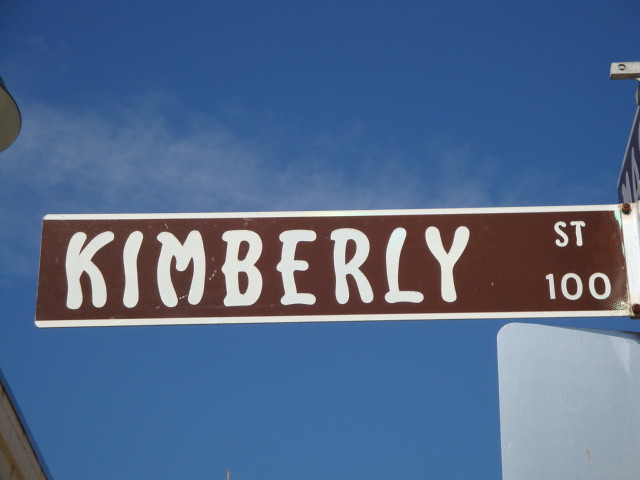The photograph prominently features a unique street sign for Kimberley Street, located in the 100 block. The sign stands out with its dark brown background and white trim, displaying the street name in a fanciful, almost cartoonish typeface, unlike typical street signs. The sky behind is a strikingly deep blue with streaks of white clouds enhancing the backdrop. Additionally, the image includes the side profile of a building on the left and the rear of another rectangular sign at the bottom right corner. A small portion of what might be another street sign, possibly for Main Street, is visible in the midsection. The overall composition is marked by a clear, bright day, highlighting the distinctive Kimberley Street sign.